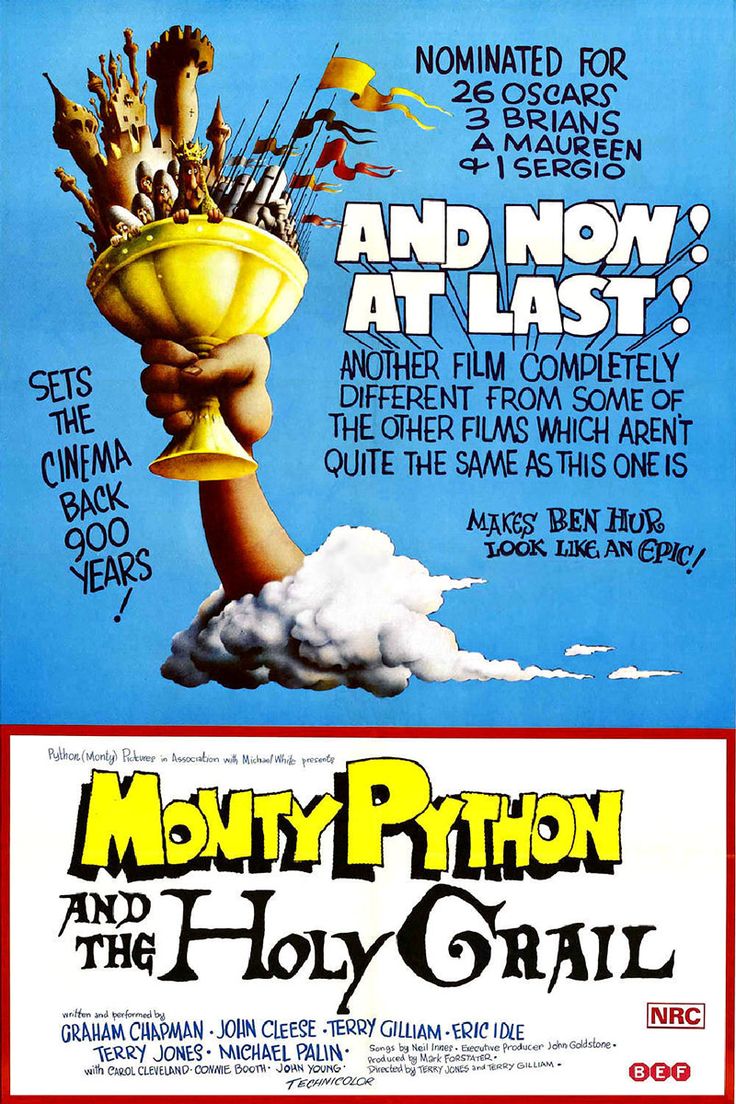The movie poster for "Monty Python and the Holy Grail" features a whimsical and detailed design. The rectangular poster, taller than it is wide, has a prominent blue upper background. Emerging from a white cloud is an arm holding a chalice. Inside the chalice, a lively castle scene unfolds with red, blue, and yellow flags, surrounded by medieval figures and creatures. Bold text on the right reads, "Nominated for 26 Oscars, Three Bryans, a Maureen, and one Sergio. And now, at last, another film completely different from some of the other films which aren't quite the same as this one, is makes Ben-Hur look like an epic." On the left, it humorously declares, "Sets the cinema back 900 years." The bottom portion of the poster features the title "Monty Python and the Holy Grail," with "Monty Python" in yellow letters and the rest in black, bordered in red. Below the title, the names of the stars—Graham Chapman, Terry Jones, Michael Palin, John Cleese, Terry Gilliam, and Eric Idle—are listed, alongside abbreviations "NRC" and "BEF," adding to the poster's playful and extravagant appeal.